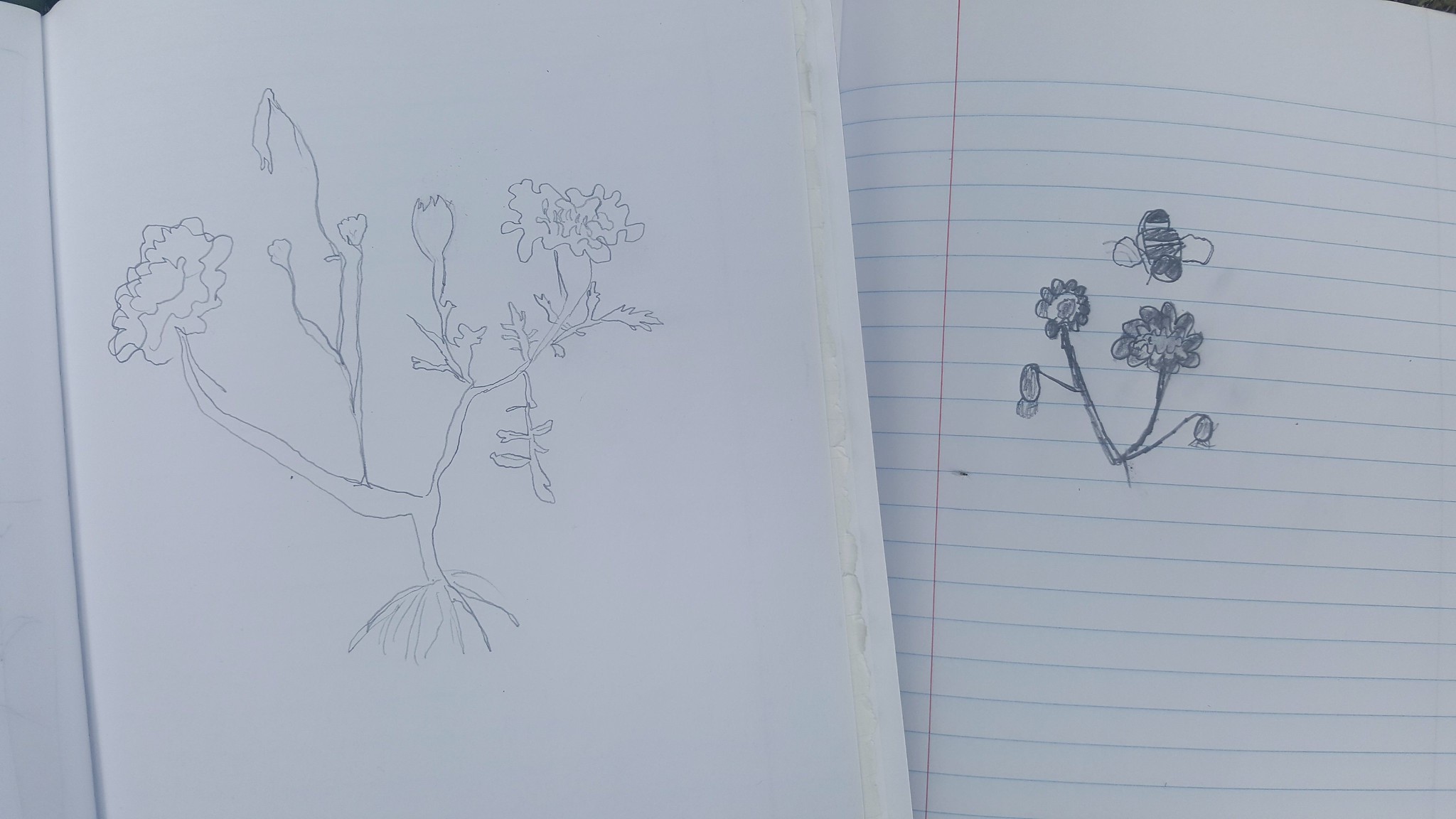In the first image, rendered with pencil on pristine white paper, we observe a detailed sketch of a pulled plant, possibly a weed or a marigold. The illustration depicts the plant uprooted, exposing its intricate root system. The stems, characterized by their rustic and irregular lines, ascend to reveal coarsely detailed leaves that branch out from the central stalk. On either side of this stem, the plant boasts a Warbledee flower, adding a focal point to the rough but expressive drawing.

Adjacent to this, the second image is a charming child's drawing on lined notebook paper, easily identifiable by its horizontal blue lines and a vertical red margin line to the left. This whimsical artwork features two simplistic, yet endearing flowers. Above them hovers a scrunkly bee, distinguishable by its quirky form and the addition of two little wings on each side, contributing to the innocence and playful nature of the image.